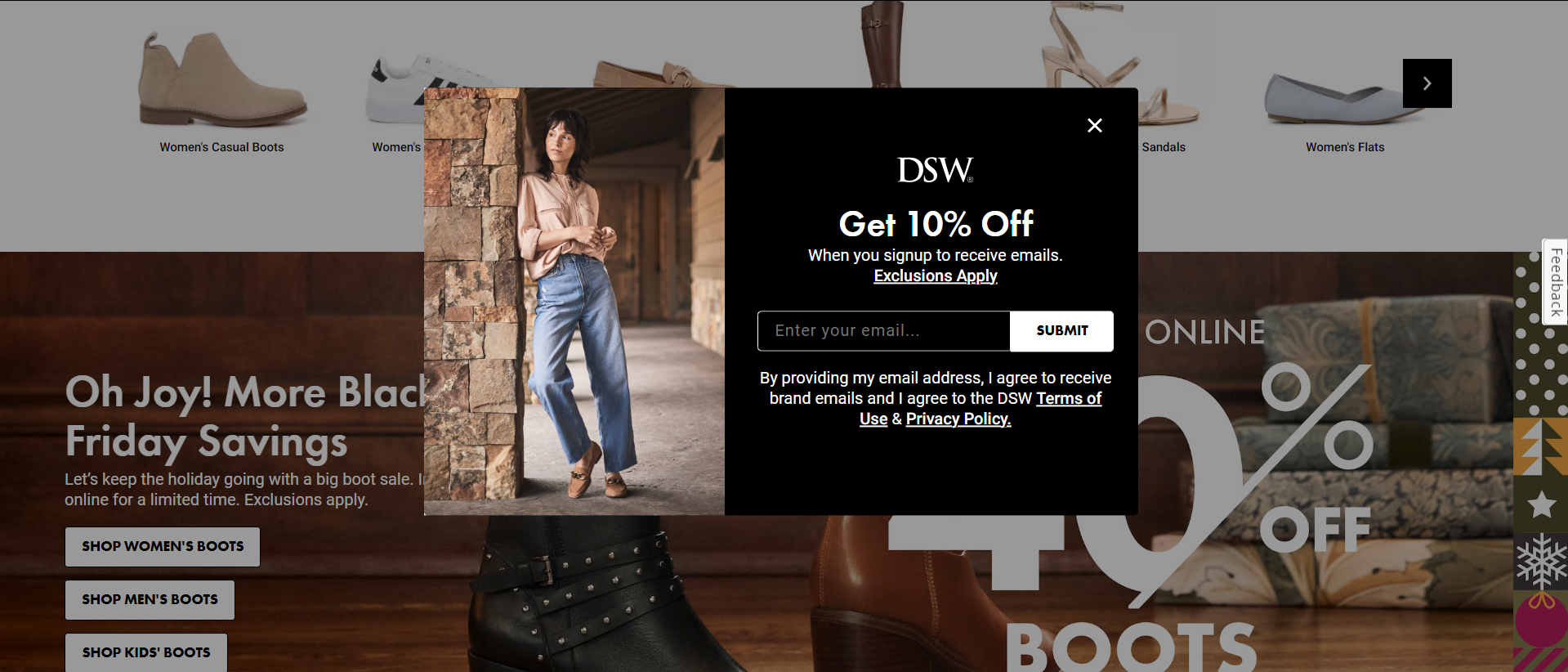The image is a promotional screenshot from DSW highlighting their Black Friday savings. At the top, there is an advertisement banner displaying a 40% discount on boots for online shoppers, with the phrase "Oh Joy, More Black Friday Savings." Below the banner are three gray rectangles with options to shop for women's boots, men's boots, and kids' boots.

To the right side, a woman is depicted wearing a pink-colored shirt, blue jeans, and tan-colored flat shoes. 

Additionally, there is a promotional offer stating "Get 10% off when you sign up to receive emails." Below this, it mentions "Exclusions Apply" which is underlined, followed by an input box to enter an email address and a "Submit" button in a white rectangle with black text. At the bottom, it includes a disclaimer that reads, "By providing my email address, I agree to receive brand emails and I agree to the," likely indicating terms and conditions.